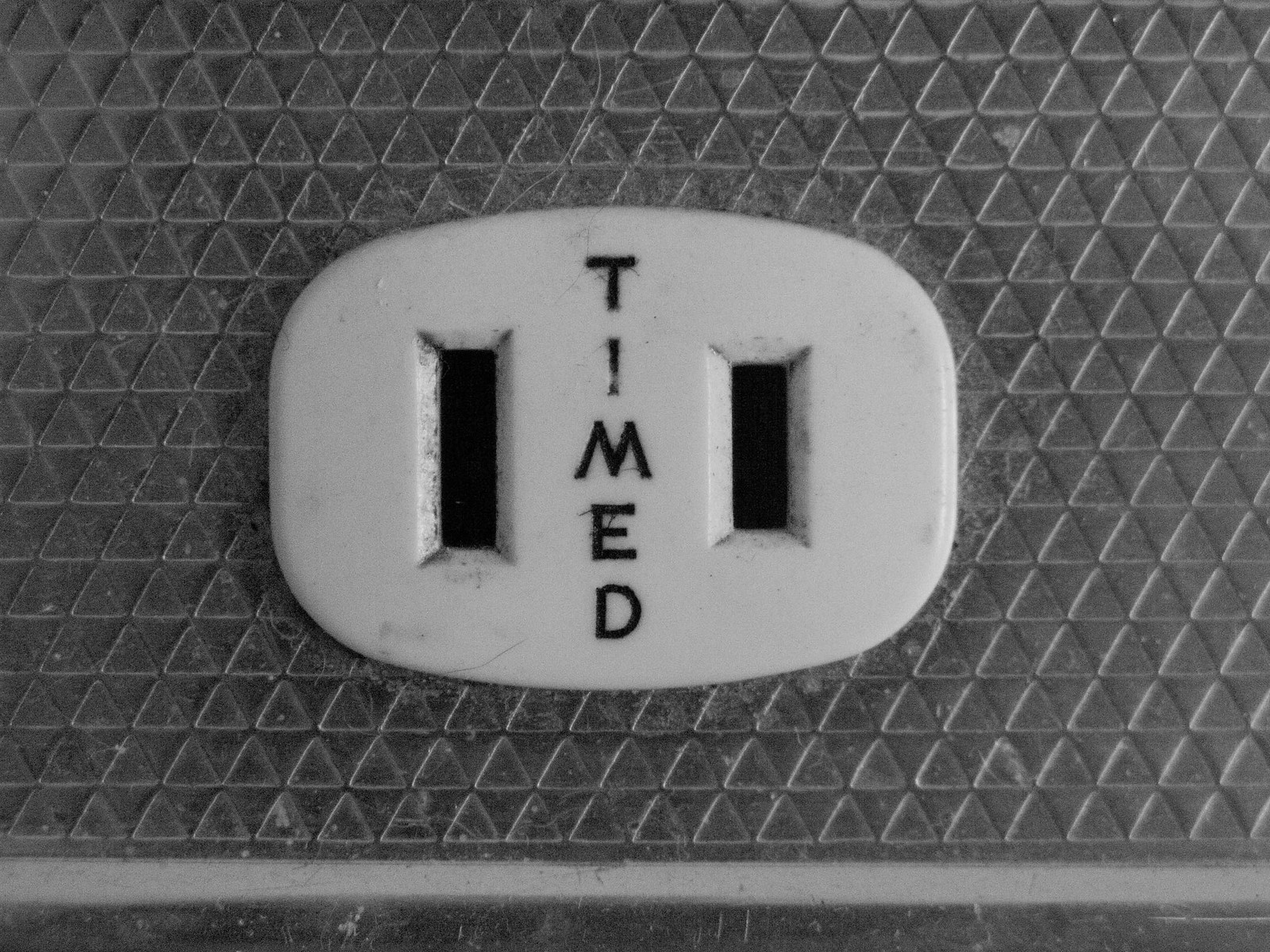This image displays an old, heavily used electrical wall receptacle marked with the word "TIMED" in the center. The receptacle features a non-grounded, American-style outlet with only two slots, characteristic of outdated electrical designs. Notably, one slot is longer than the other, a common feature in older U.S. plugs. The wall surrounding the receptacle is adorned with triangular patterns, evoking an aged or possibly retro aesthetic, reminiscent of what one might find in an old motel or similarly outdated building. This type of outlet, lacking the modern third, grounding prong, has fallen out of standard use in favor of safer, updated designs.